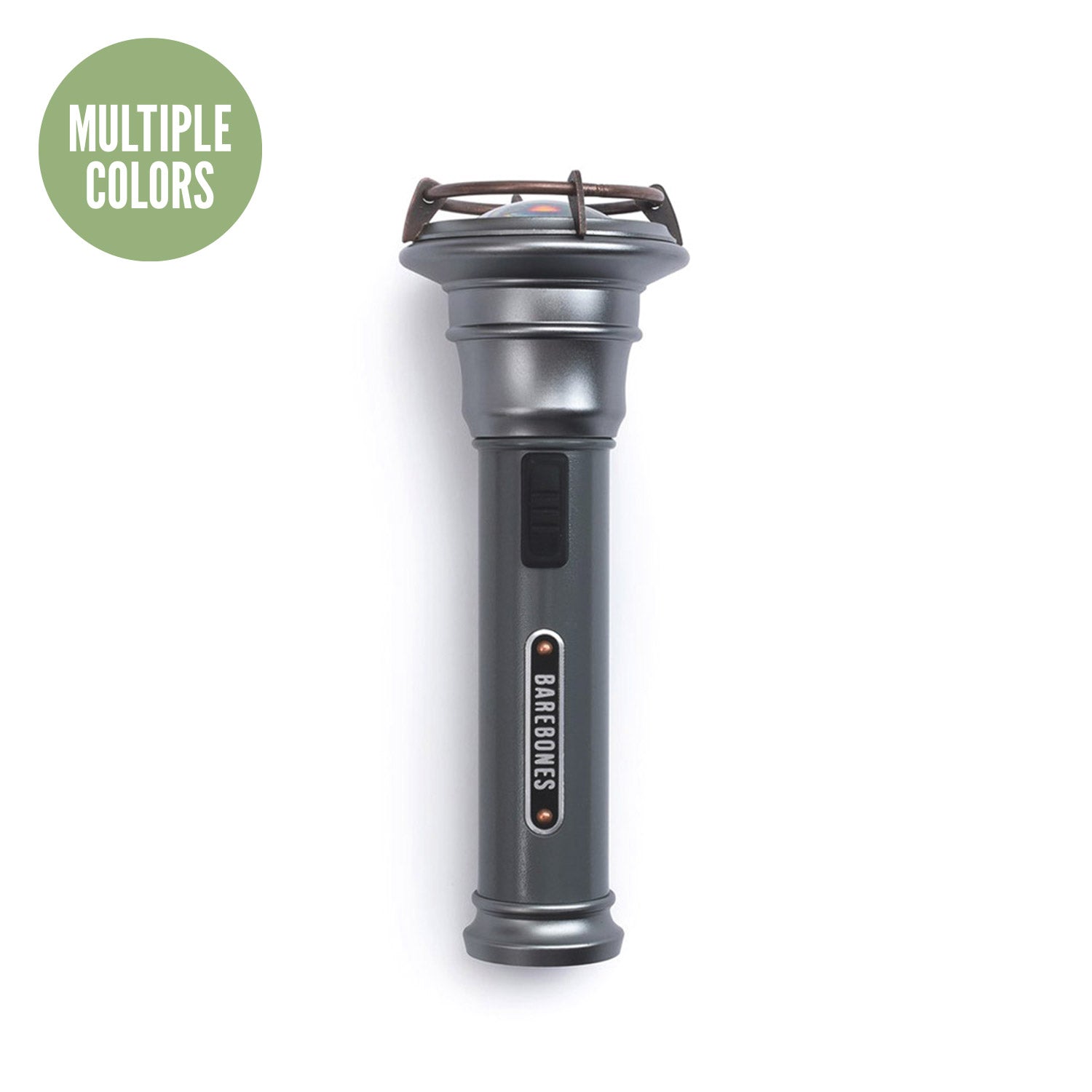This is a professionally taken photograph featuring a sleek, cylindrical, battery-operated flashlight from Barebones, depicted against a pristine white background. The flashlight is predominantly silver with a charcoal hue, complemented by a black switch on its body. A prominent black oval with white capital letters spelling "Barebones" adorns the side. Flanking the logo are light gold circular buttons. The upper section of the flashlight, encased in a protective brown railing, houses a covered light source that emits a subtle orange glow, indicating it may be illuminated. Floating in the upper left corner of the image is a pea green circle with white capital letters announcing "Multiple Colors," suggesting that the flashlight is available in various color options. The photograph emphasizes the tool's high-tech, sophisticated design, ensuring viewers get a clear and detailed understanding of its appearance and features.